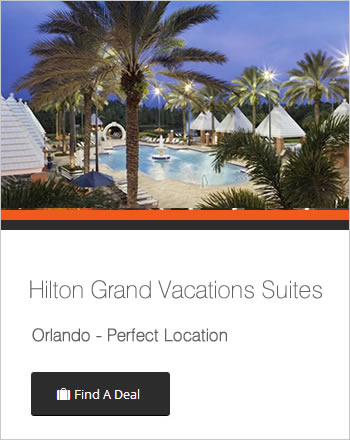This screenshot features the Hilton Grand Vacation Suites located in Orlando, Florida, captivating viewers with its luxurious resort-style ambiance. Central to the image is a stunning pool area, adorned with graceful palm trees and cozy cabanas perfect for relaxation. Bathed in the warm, soothing glow of evening lighting, the scene exudes a tranquil atmosphere. The image also includes a prominent call-to-action button labeled "Find a Deal," suggesting an enticing opportunity for affordable rates, ideal for those looking to make reservations or explore offers at this opulent destination. The harmonious blend of promotional text and imagery underscores the appeal and accessibility of this prime vacation spot.